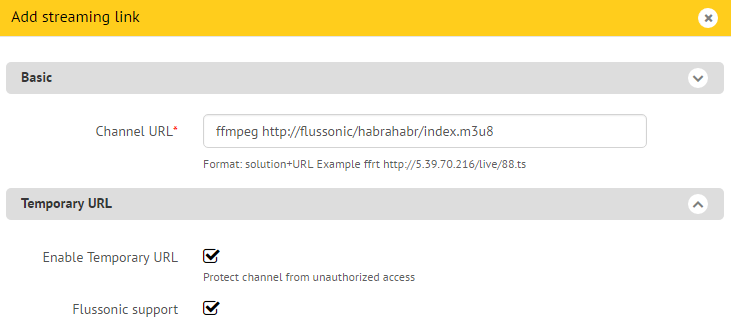The top section features a yellow bar with "Add a Streaming Link" written in black text on the top left corner. In the top right corner of the yellow bar, there is a small white circle containing a gray X. The rest of the page is predominantly white, interspersed with gray bars. 

The first prominent gray bar displays "Basic" in bold black text on the left side, accompanied by a small white circle with a downward-facing gray arrow on the right side.

In the white section below, "Channel URL" is labeled with a red asterisk. There is a white text box beneath this label, containing the URL: "FFmpeghttp://fluasonic.havrabar.index.m3u8". Following this, there is information labeled "Format," including a section titled "Solution + URL Example" which provides an example URL.

Another gray bar below this section is labeled "Temporary URL" and features a small white circle with an upward-facing arrow. Further down, two checkboxes offer the following options: "Enable Temporary URL" and "Fluasonic Support." The first checkbox also includes a specific option to "Protect Channel from Unauthorized Access."